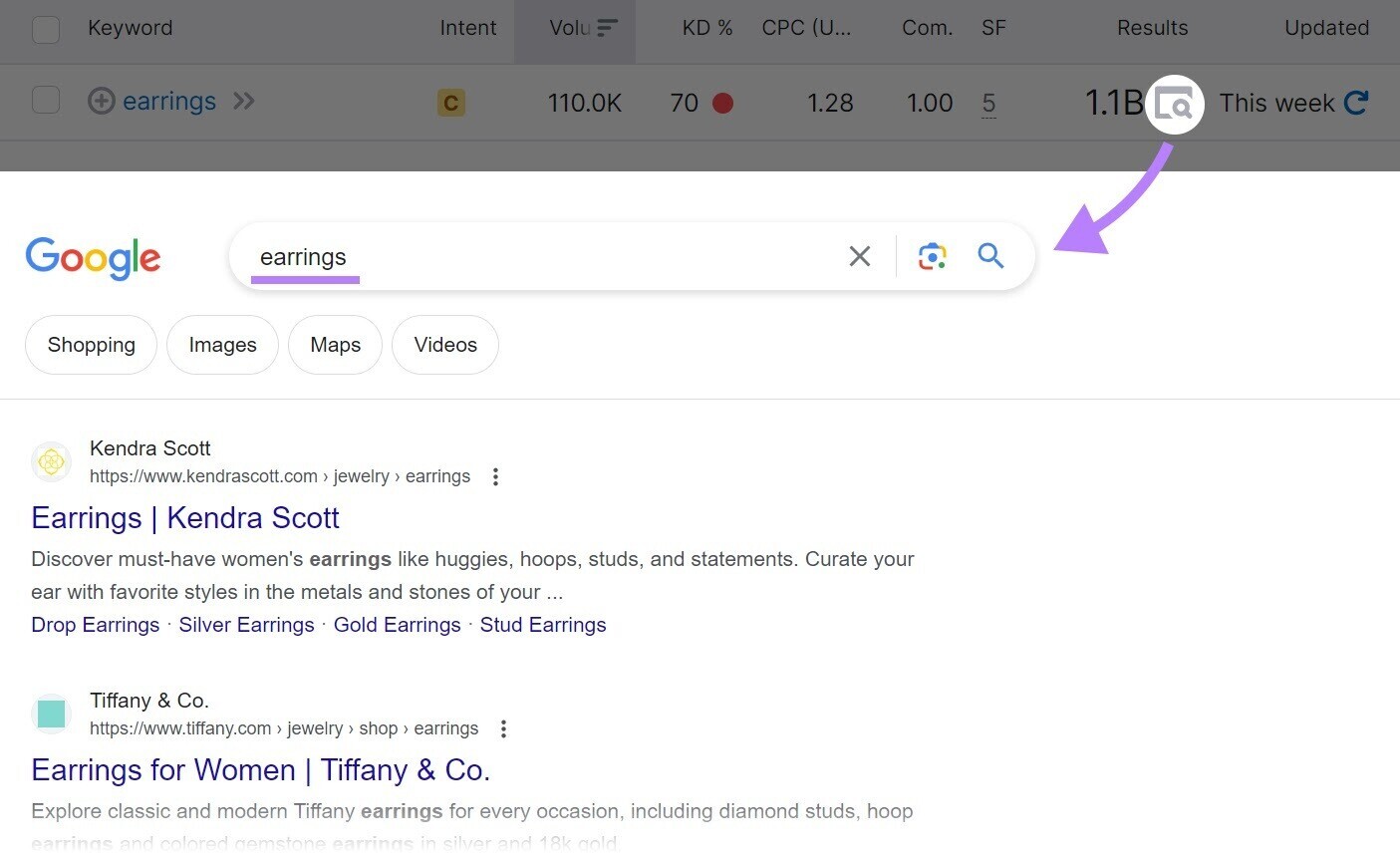In the image, we see a Google search results page. The search query "earrings" is prominently displayed, highlighted by a distinctive purple bar beneath it. Below this bar, a horizontal menu offers various categories like Shopping, Images, Maps, and Videos.

The first search result is a link to Kendra Scott earrings, presenting a preview text that reads: "Discover must-have women's earrings like huggies, hoops, studs, and statements. Curate your ear with favorite styles and the metals and stones of your...". Additionally, there are sub-sections for various earring types such as drop earrings, silver earrings, gold earrings, and stud earrings.

The second link directs to Tiffany & Co., featuring a caption: "Earrings for women, Tiffany & Co. Explore classic and modern Tiffany earrings for every occasion, including diamond studs, hoop earrings, and colored gemstone earrings in silver and 18-karat gold."

At the top of the page, there's a grayed-out section with a purple arrow pointing to an icon. This section elaborates on various metrics related to the search term "earrings," including intent, search volume, keyword difficulty (KD), and cost per click (CPC). This section is shown in a gray box, providing additional context if the icon were clicked.

Overall, the image effectively showcases a Google search interface focused on the term "earrings," detailing popular brands and types, while offering useful metrics for search optimization.